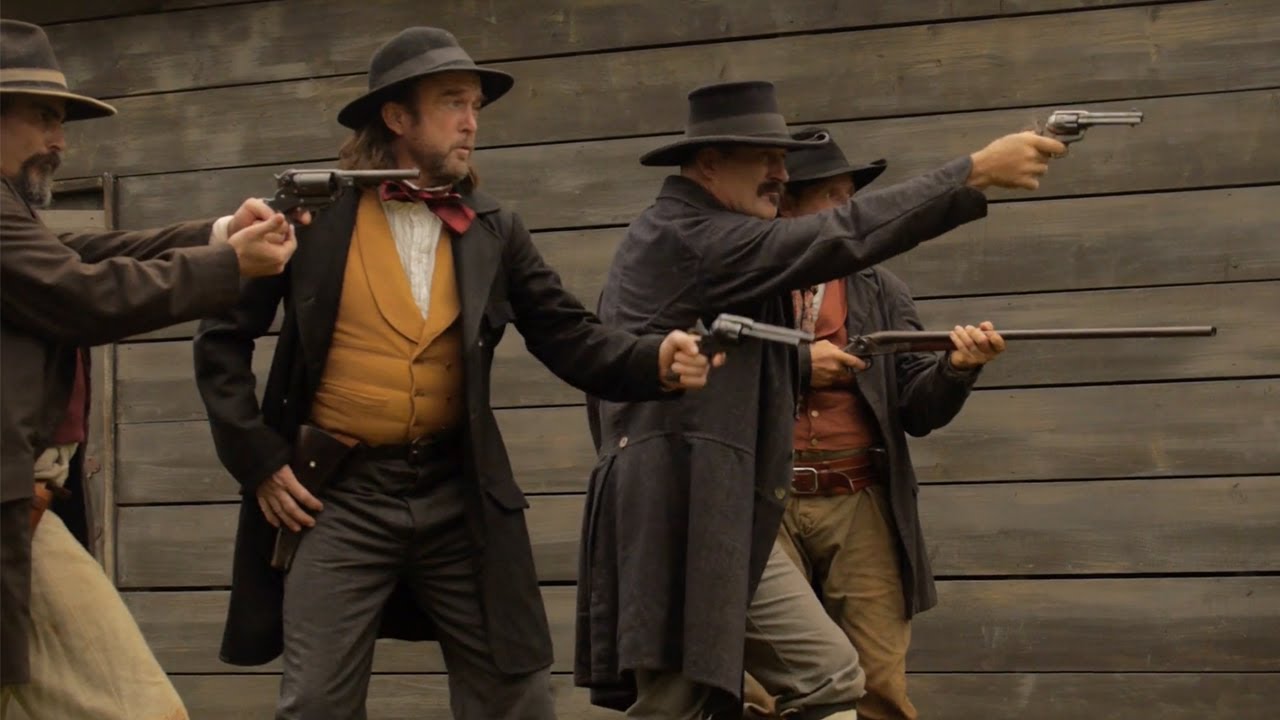This image, likely a screenshot from a Western movie or a reenactment at a Wild West theme park, captures four gentlemen in period-appropriate attire. They are all intently focused to the right, with their weapons drawn, suggesting a standoff or confrontation scene. The background features wide, dark wooden slats resembling the side of a building. 

The man closest to the viewer is partially visible, dressed in white pants, a brown coat, and a brown hat with a light brown stripe. He sports a goatee and wields a rifle. Next to him, the second man stands with one hand on his hip, wearing a bright yellow vest, a brown coat, brown pants, and a brown hat. He has longish brown hair, a beard, and appears to be sporting a red bowtie while holding a black pistol. 

The third man is dressed in all brown, including his hat, and has a mustache. He holds a silver pistol in his right hand. The fourth man, positioned furthest back, holds what appears to be a shotgun. He is attired in a reddish-orange vest, a dark jacket, and brown pants.

Each man exhibits a stern expression and poses in a slight crouch, ready to shoot, enhancing the tension and drama captured in this vivid, striking image.